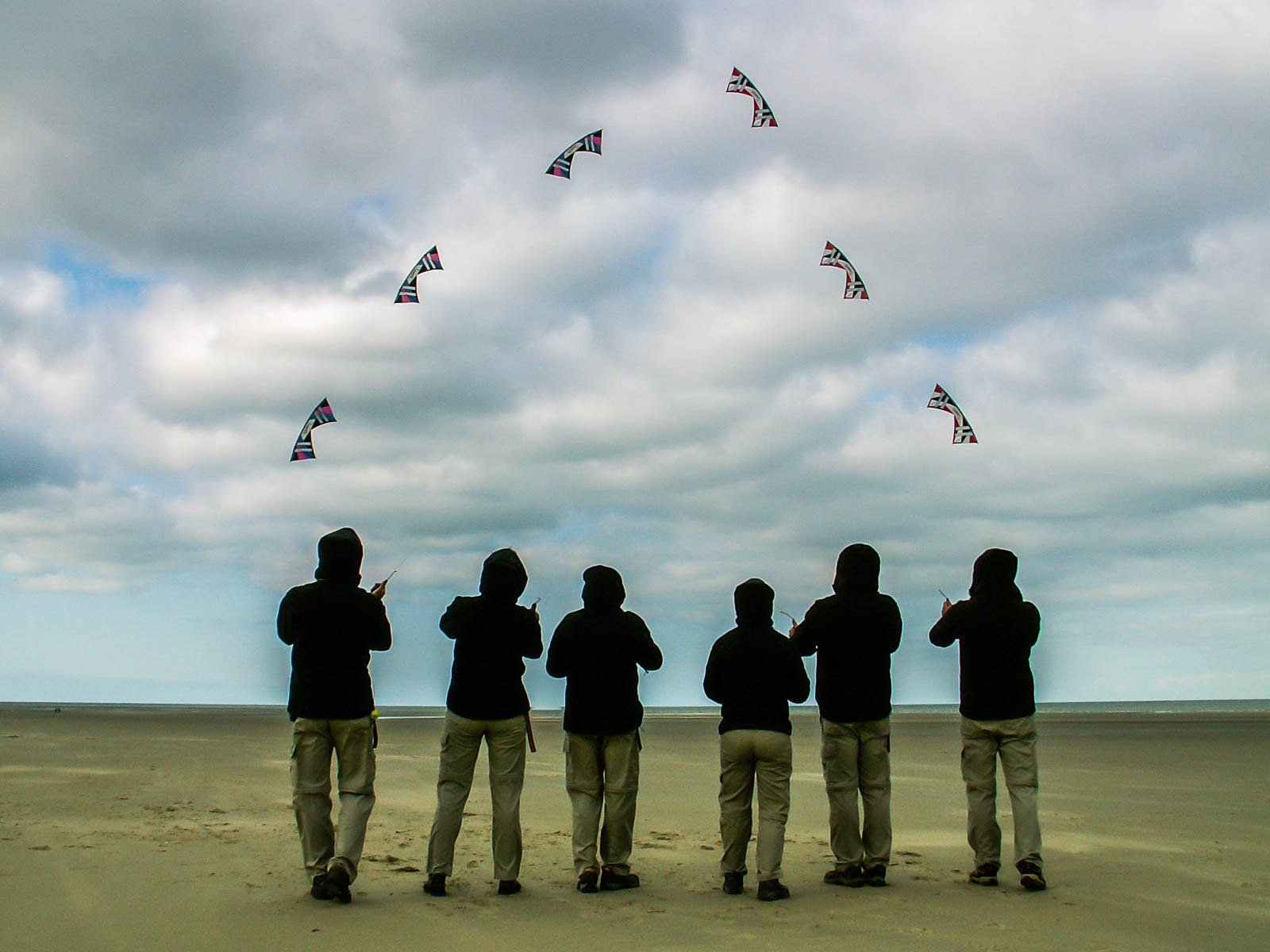In this outdoor photograph, six people stand close together on a sunlit, compacted dirt field, their backs facing the camera. Each person wears a black hoodie, khaki or camouflage pants, and black shoes. The group is depicted flying kites, each adorned in red, white, blue, and black colors, patterned to resemble stylized birds rather than national flags. The kites are arranged in a loose triangular formation in the sky, which is a rich blue, adorned with fluffy white and gray clouds, adding a picturesque backdrop to the scene. The horizon appears to meet either the ocean or a vast expanse, further emphasizing the openness of their surroundings.